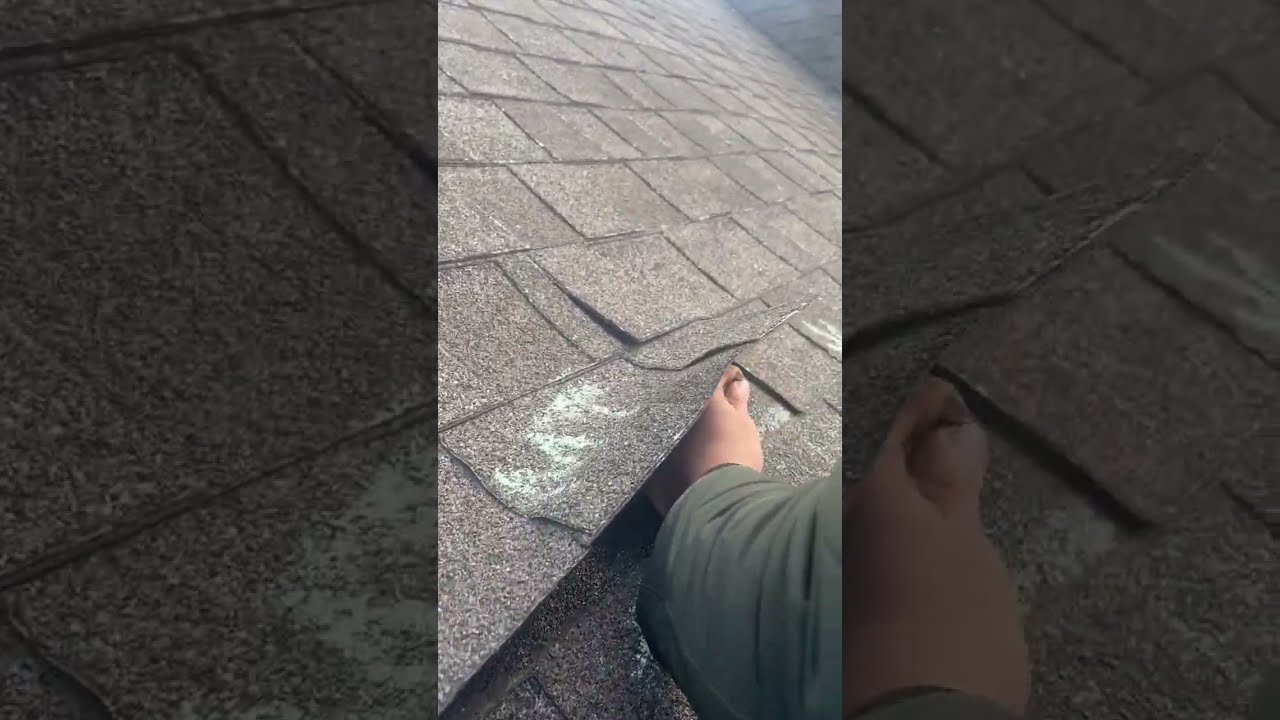The image depicts a close-up view of a rooftop shingling process, seen from the perspective of someone standing on the roof during the day. In the center of the horizontal rectangle photo, a person's arm, clad in a gray long-sleeve shirt, extends from the bottom right corner, holding a nail and lifting a roof shingle. The tiles, oriented diagonally from the camera's viewpoint, show signs of wear, revealing the base material beneath the asphalt layer. The focus emphasizes the hand and the roofing task, while, in the upper right corner, another section of the roof is barely visible, indicating an intersection of two roof planes. The image is surrounded by wide borders on both the left and right sides.